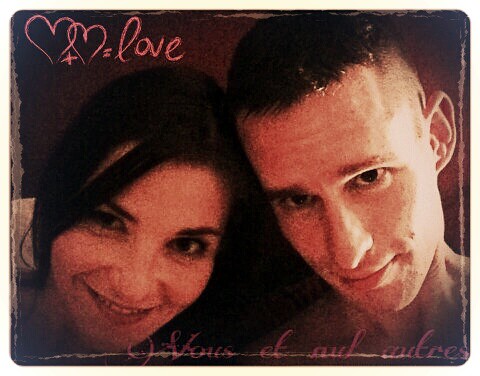A photograph of a young couple shows their heads tilted towards each other, smiling warmly at the camera. The woman, positioned on the left, has dark brown hair cascading down around her face, with expressive dark eyes and a beaming smile. The man, on the right, displays short brown hair with shaved sides and a slightly longer top, accompanied by a subtle smirk and a need for a shave. They appear very close, almost touching heads, capturing a moment of shared joy. In the top left corner, a handwritten pink graphic features two hearts connected by a plus sign, an equal sign, and the word "love". The photograph, seemingly a picture of a worn physical photo, is slightly grainy and shows signs of wear around the edges, suggesting it was once in a frame. At the bottom, there is some faint pink cursive writing, possibly in French, which is difficult to read due to its light coloration and blurriness.